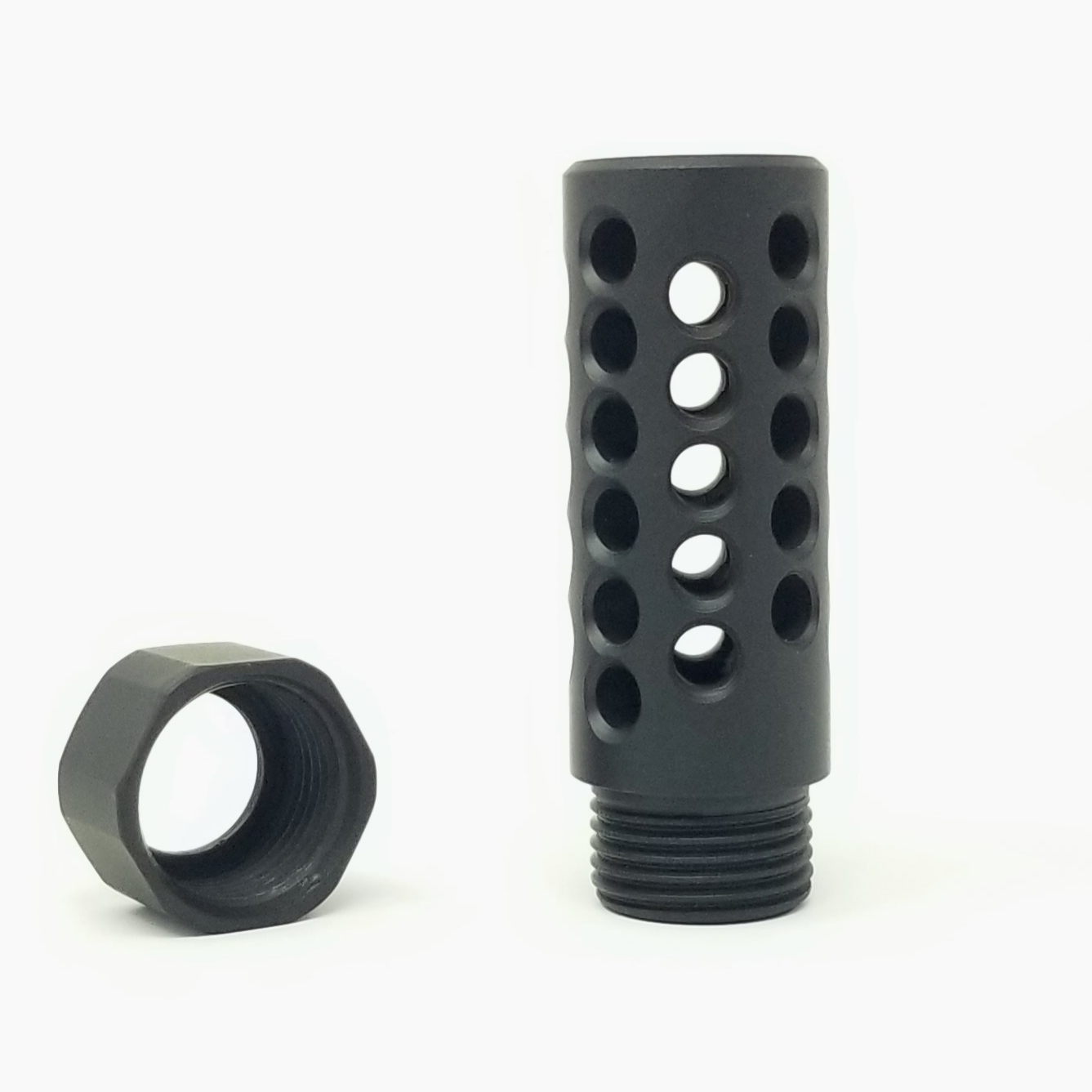The photograph features a product placed on a completely white background. The central object is a black cylindrical bolt, which appears hollow and is perforated with evenly spaced holes along its length. These perforations allow the white background to be visible through the cylinder. The bottom end of the cylinder is threaded, suggesting it can be screwed into another part. To the right of the bolt, there is a hexagon-shaped nut, matching the diameter of the threaded section of the cylinder. This nut also has an internal thread that would allow it to screw onto the bolt. The overall purpose of this item is not indicated, but it may serve as an attachment or component for machinery, such as a pressure washer. The precise spacing and number of the perforations, with six on the left side, five in the middle, and five on the right, highlight the even distribution and uniform design of the bolt.